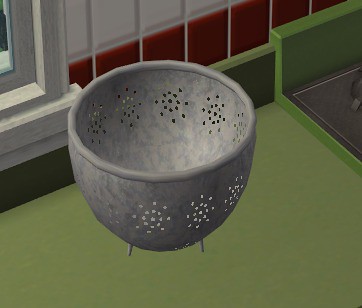In this image, we see a detailed 3D model of a bowl-like object, possibly made of copper or another metallic material. The bowl is adorned with numerous intricate cut-out patterns resembling little flowers. The bowl is circular at the top, transitioning to a more oval shape at the base, supported by two small grey legs. It has a sun-like design on its surface, adding to its artistic appearance. The bowl is situated on a green surface, which seems to be elevated slightly above a grey floor area. The background includes white and red square-tiled walls, with the red tiles at the bottom separated by white grout. In the top right corner, there is an unclear grey flat surface. Additionally, to the left in the background, a white windowsill or picture frame is partially visible. The overall environment appears to be designed in a somewhat pixelated, cartoony style, suggesting it might be from a digital or gaming context.